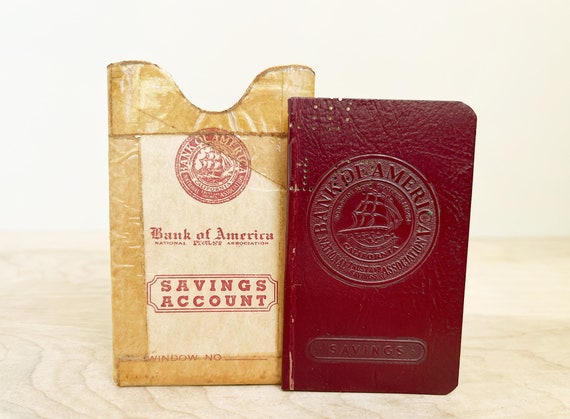The photograph features a set of vintage banking items placed against a light, possibly white or pink, background with subtle patterns near the bottom. Centered on a light wooden table are two meticulously detailed objects: an old savings account book and its protective cover. On the left is a yellowed cover with the Bank of America logo prominently displayed at the top. Beneath the logo, the words "Bank of America, Savings Account, Window Number" are crisply printed in red. The cover is noticeably aged, with cellotape repairs and scratch marks. To the right is a deep red passbook, embossed with "Bank of America, National Trust and Savings Association." The passbook also features an oval stamp showing a ship and the word "Savings" below it, emphasizing its status as a historic savings account book. Both items evoke a sense of nostalgia and reflect the meticulous banking practices of yesteryear.